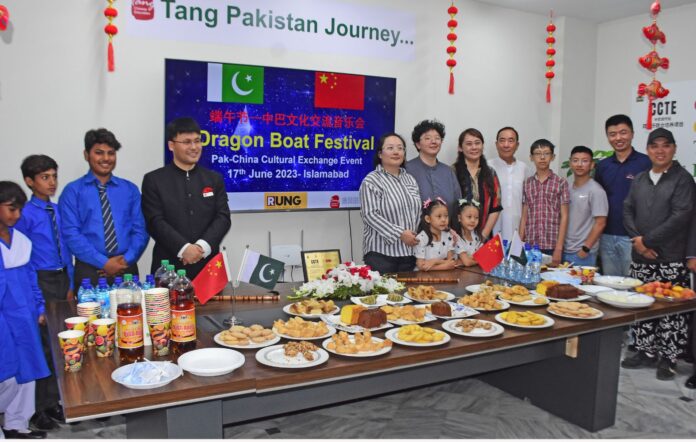This amateur photograph captures a vibrant cultural exchange event between Pakistanis and Chinese individuals, held on the 17th of June, 2023, in Islamabad. The foreground is dominated by a long table laden with a variety of dishes, white plates, cups, and bottles containing red beverages, hinting at a small feast. In the middle of the table, a floral centerpiece adds a touch of elegance.

The backdrop features a large TV screen displaying a blue presentation sign that marks the occasion as the Dragon Boat Festival and a Pakistan-China Cultural Exchange. The presentation includes the flags of both nations—the green and white flag of Pakistan and the red and yellow flag of China—along with the title "Tang Pakistan Journey..." displayed on a printed banner. Traditional Chinese decorations, such as red lanterns and decorative strands with fish and tassels, adorn the room, enhancing the cultural ambiance.

The photograph depicts 14 people, with four individuals standing on the left and a larger group on the right. The attendees, including children, are mostly dressed in modern Western attire. The mixture of people—predominantly of Asian descent—reflects the friendly and communal spirit of the cultural exchange event.